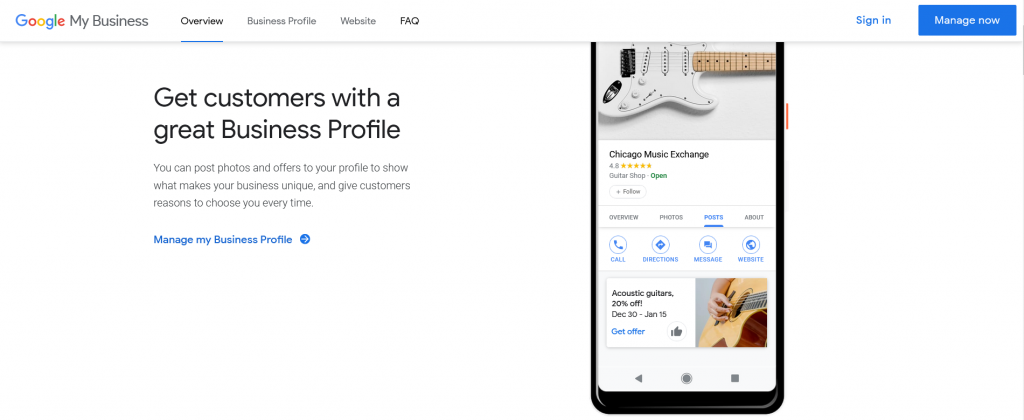The image features a predominantly white background with the word "Google" prominently displayed in the upper left-hand corner, indicating the business brand. The letters of Google are color-coded: the first letter is blue, the second is red, the third is yellow, the fourth is blue again, the fifth is green, and the final letter is red. Below "Google," the text "My Business" appears in black font.

The interface shows several tabs aligned horizontally. The first tab, labeled "Old You," is bold and underlined in blue, signifying the active tab. Other visible tabs include "Business Profile," "Website," and "FAQ," along with additional frequently asked questions. Below this navigation bar, there is more content spaced out.

In black text, a heading reads, "Get Customers with a Great Business Profile." In a slightly smaller font, further guidance is provided: "You can post photos and offers to your profile to show what makes your business unique, and give customers reasons to choose you every time." 

Beneath this instructional text, a blue button reads "Manage My Business Profile." Adjacent to the button is a blue circle featuring a white arrow.

The remaining visible portion of the interface shows a partially cut-off image of a white electric guitar. Below this image, the text reads "Chicago Music Exchange" in black, followed by a rating of "4.8 out of 5 stars." The business category "Guitar Shop" is listed in gray, and its operational status, "open," is displayed in green.

Further tabs beneath the business information include "Overview," "Photos," "Posts" (highlighted in blue), and "About." Additional action buttons in blue text read "Call," "Directions," "Message," and "Website."

At the bottom, a promotional message in black announces, "Acoustic Guitars, 20% off December 30th through January 15th." A blue "Get Offers" button is also visible.